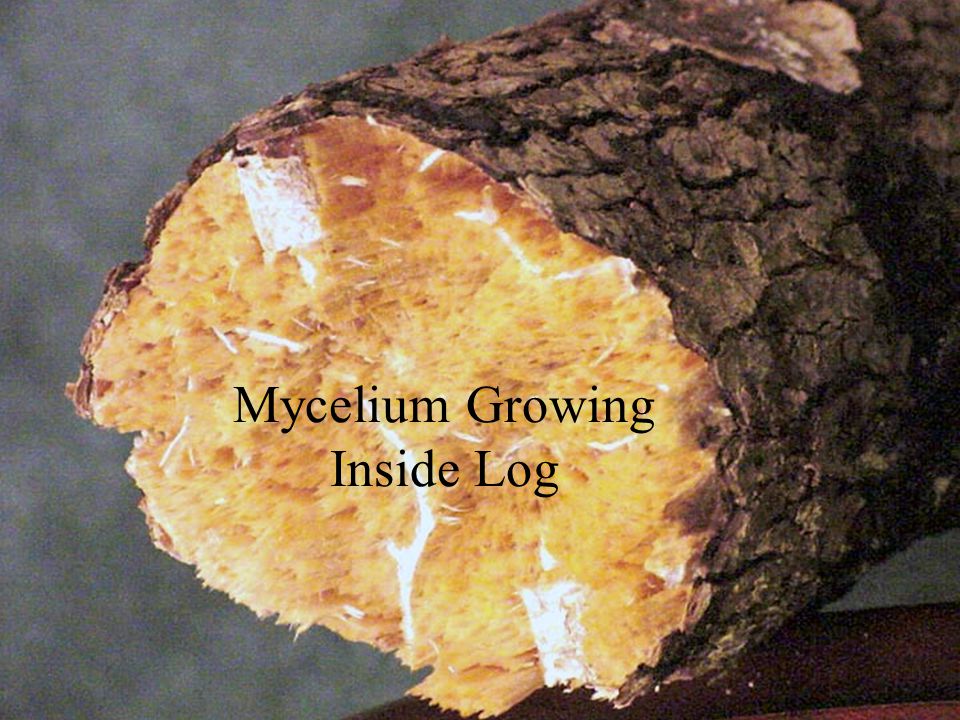The image features a close-up shot of a cut log, positioned against an abstract, blurry grey background. The camera is pointed towards the cut end of the log, which shows a section of its interior and exterior. The interior of the log reveals a yellowish or light brown wood, colonized by patches of white mold, likely mycelium, as indicated by the text superimposed on the image that reads "Mycelium growing inside log." The rough exterior surface of the log is still clad in dark brown bark, exhibiting various ridges and natural divisions. The log extends from the center of the image towards the top right corner, and it appears to be resting on a wooden table.